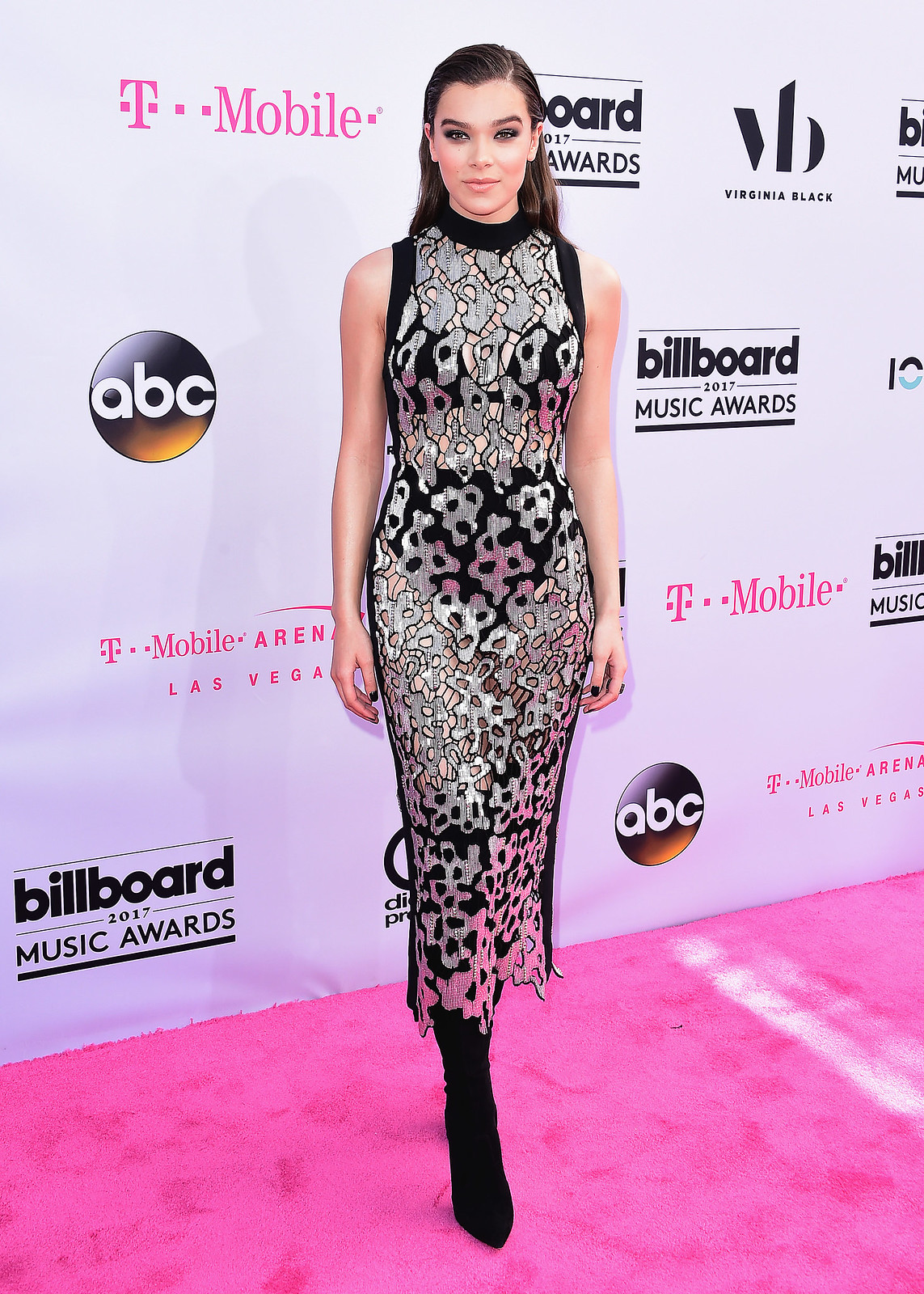This photograph, likely taken at the 2017 Billboard Music Awards, features a young woman posing on a vibrant, bright hot pink carpet. The backdrop is a white wall adorned with various repeated logos including T-Mobile, ABC, Billboard 2017 Music Awards, and Virginia Black. The woman, who appears to be a celebrity, is showcasing a fancy, eye-catching sleeveless dress with a gold, black, and silver trippy pattern that has a slight see-through sheen in parts. She has long brunette hair, styled straight and pulled back behind her shoulders. Her outfit is complemented by high-heeled black boots which extend up her legs, with her right boot positioned forward, subtly obscuring her left foot. She is looking directly at the camera with arms resting by her side and giving a slight, closed-mouth smile.